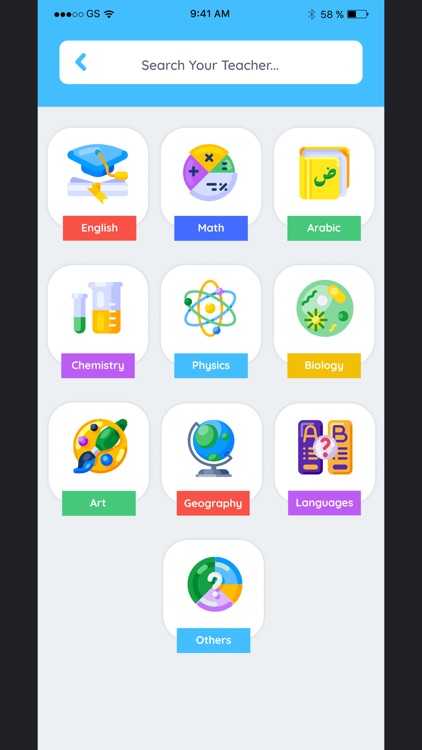The image appears to be a screenshot or a photograph of a smartphone screen. The screen has black edges along the left and right sides. At the top, there is a blue background displaying the status bar. On the left side of the status bar, you can see the Wi-Fi symbol. In the center, the time is displayed as 9:41 AM. On the right side, it shows the battery percentage at 58%.

Below the status bar, there is a large white search box with the text "Search your teacher." Beneath the search box, there are a series of app icons arranged in a grid layout. The icons are small, rounded white squares, each containing a different image and corresponding text.

The first row contains three icons:
1. The first icon is a white square with an image of a graduation cap and a diploma, labeled "English" in a red rectangle.
2. The second icon is a white square depicting a test tube and a beaker filled with liquid, labeled "Chemistry" in a purple rectangle.
3. The third icon is not described.

The second row contains three icons, but only the third icon from the first row is specifically detailed.

The third row also contains three icons, but again, only the first icon is detailed:
- It features a white square with an image resembling a paint palette and a paintbrush, labeled "Art" in a green rectangle.

The fourth row has a single icon centered on the screen. 

Overall, the image shows a neatly organized user interface of a smartphone screen, possibly an educational app or portal, featuring various subject icons for easy access.